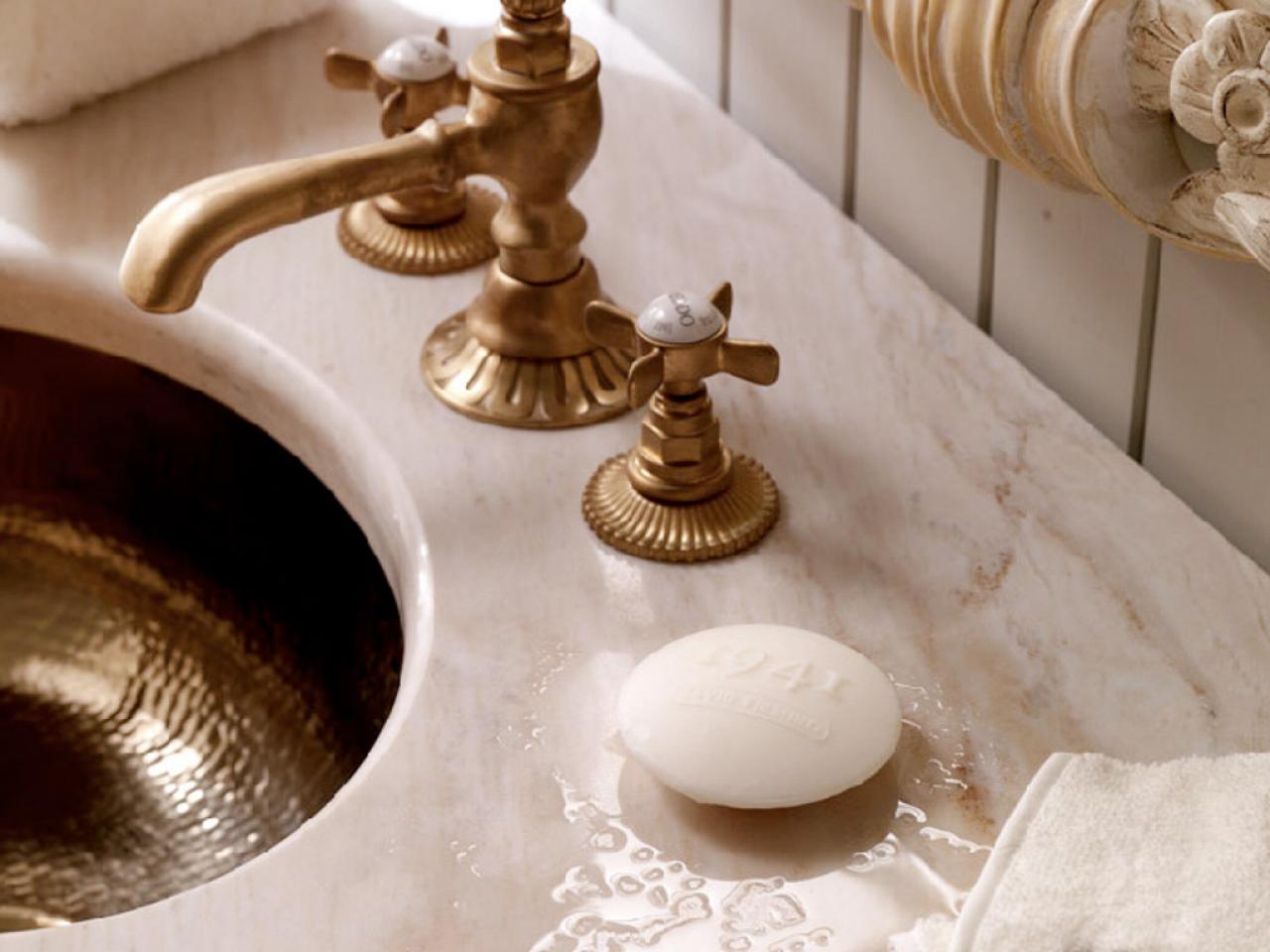This close-up image displays a bathroom sink with a light gold, rippled basin set into a marble countertop of a light pinkish hue with visible water splatters. The faucet and handles are a copper or gold color with white caps. There’s a bar of soap on the right knob, inscribed with "1941" and other illegible text. Two white towels are in the image - one in the top left corner and another in the bottom right. The background features white tiles with gray lines and a decorative white and beige piece in the top right. The image is high quality, illustrating the sheen of the marble countertop and the subtle wear on the decorative piece.